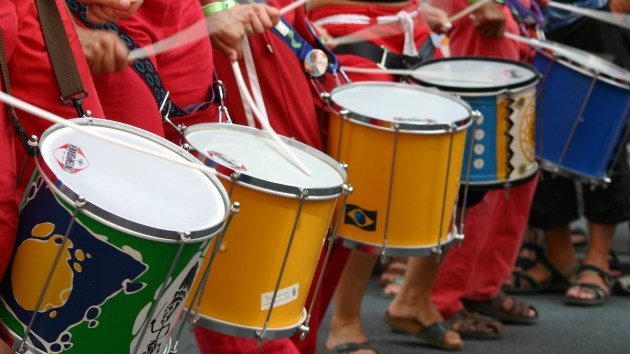This color photograph captures a vibrant scene of a drumline mid-performance, possibly during a parade. Focusing on the drums worn by five drummers dressed in striking red outfits, the image only reveals the musicians from the waist down, emphasizing their uniform red pants and brown leather sandals. Each drummer holds drumsticks and is actively drumming on snare drums secured by harnesses.

The composition highlights a row of five snares, each with distinct, colorful designs. Starting from the lower left corner, the first drum is green with blue and yellow accents. The next two drums are solid yellow, while the fourth drum showcases a combination of blue, white, and gold. The line concludes with a solid blue drum accented with white. Every drum features a white top and a silver frame, creating a cohesive yet diverse visual. The dynamic scene exudes an energetic rhythm and suggests a lively, coordinated performance by the red-clad drummers.